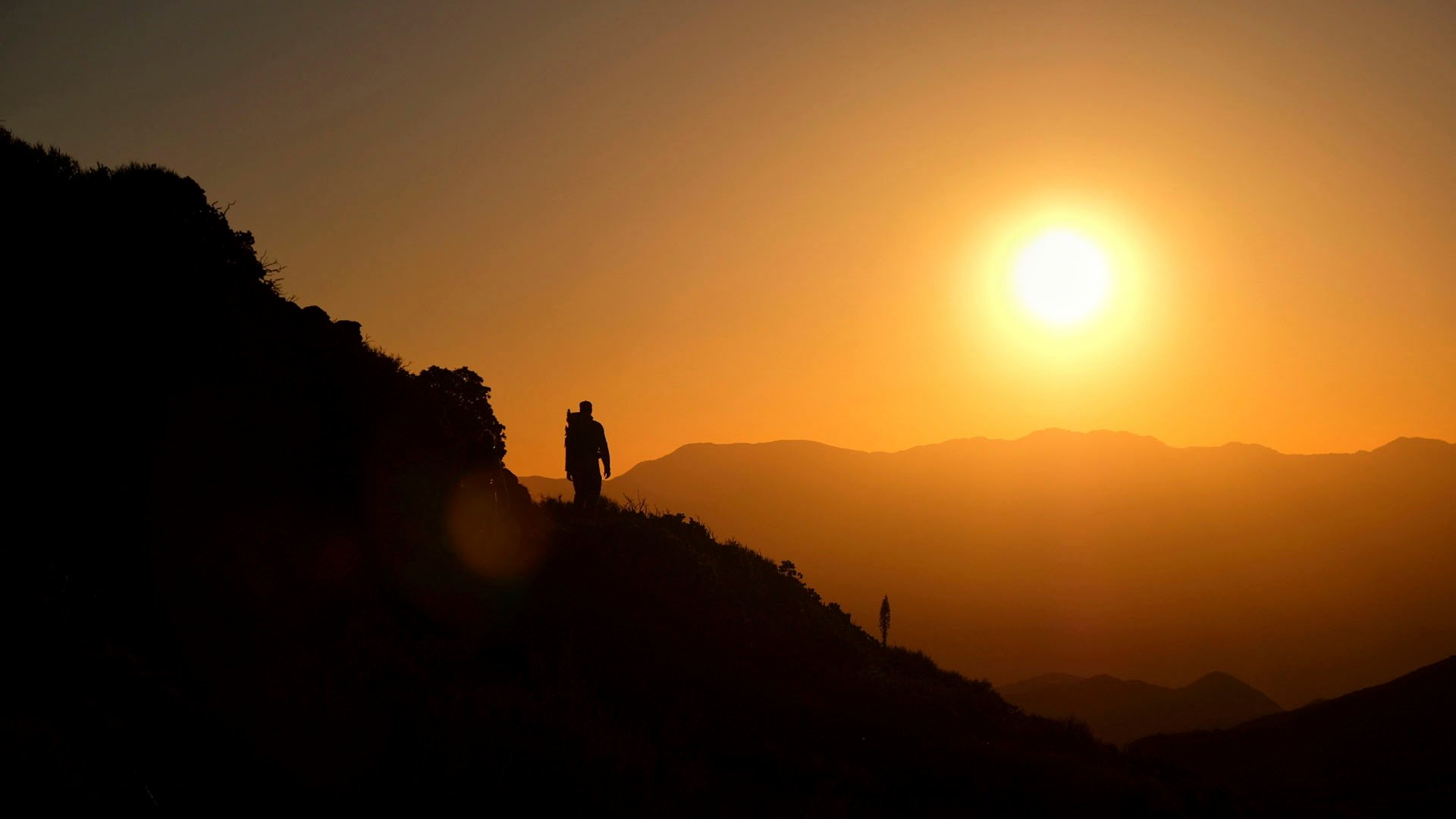In this breathtaking photograph, two hikers are silhouetted against the setting sun as they navigate a rugged, downward-sloping mountain. The closest hiker, identifiable by a backpack, stands out starkly against the rich amber, tangerine, and sepia hues of the sky, indicating the end of day. Farther down the slope, a second, smaller silhouette can just be seen. The sun, a glowing white orb with radiant yellow beams, hangs low over the horizon, casting an ethereal light on the scene. The distant mountains blend into a darker orange, almost sepia, framing the serene yet rugged landscape with a sense of depth and grandeur. The terrain is clearly rough and rocky, adding to the dramatic and adventurous essence of the image.